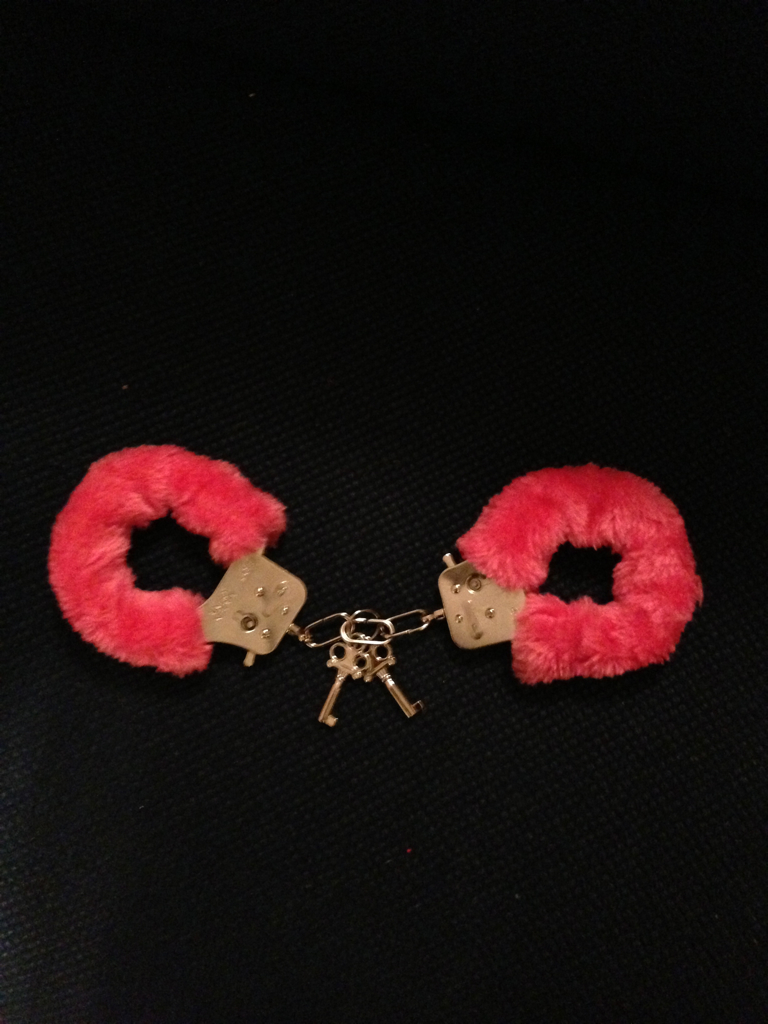The image depicts a pair of pink, fuzzy handcuffs resting on a black background, likely a tightly woven fabric akin to sofa material. The plush, vibrant pink fur covers the wrist areas of the handcuffs, giving them a warm rose hue. The metal components, including the parts where the keys go in, are in silver, featuring a few small divots. The handcuffs are spread out with a small interlocking chain connecting them. From this chain, two keys dangle, each with tiny holes at the top for easy handling. The keys have a slight gold hue, and one key points slightly down and to the left while the other points down and to the right. The overall arrangement shows the fuzzy sections of the handcuffs on the left and right, with the square-shaped lock parts tilted inward, emphasizing the central chain and dangling keys.